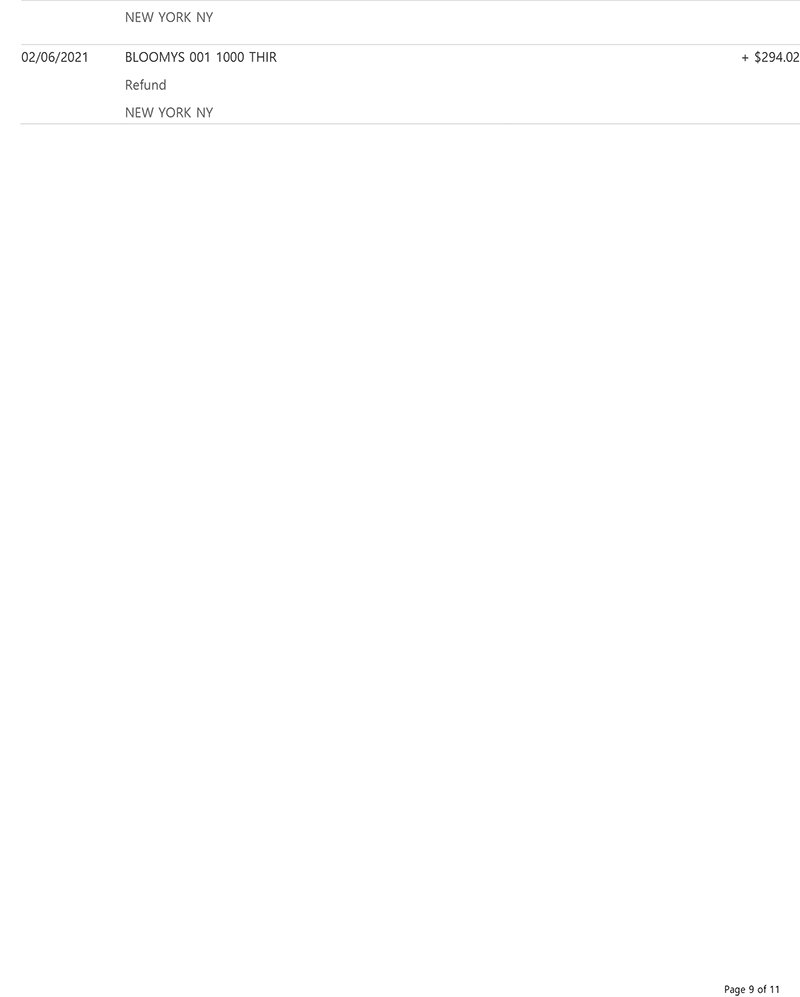A small, detailed ledger is depicted in the image. The ledger spans approximately six to eight inches horizontally and about one and a half inches vertically. The top section, comprising 20% of the ledger, features a rectangle bordered by gray lines at the top and bottom. Inside this rectangle, the text reads "New York, New York."

Beneath this, the main body of the ledger is organized in a second box. On the far left, the date "02/06/2021" is clearly written. Directly under "New York, New York" (spelled out), the entry lists "Blummies" followed by "001-1000-THIR." Below this, the term "refund" is prominently featured, with "New York, NY" restated directly underneath.

To the far right of the ledger, approximately three to four inches from the left margin, the amount "+$294.02" is noted, indicating a dollar amount with a preceding plus sign. Finally, at the bottom of the ledger, the text "page 9 of 11" is visible, though it appears to be somewhat disconnected from the detailed entry described above. This ledger entry documents a refund from "Blummies" in New York, NY for $294.02.